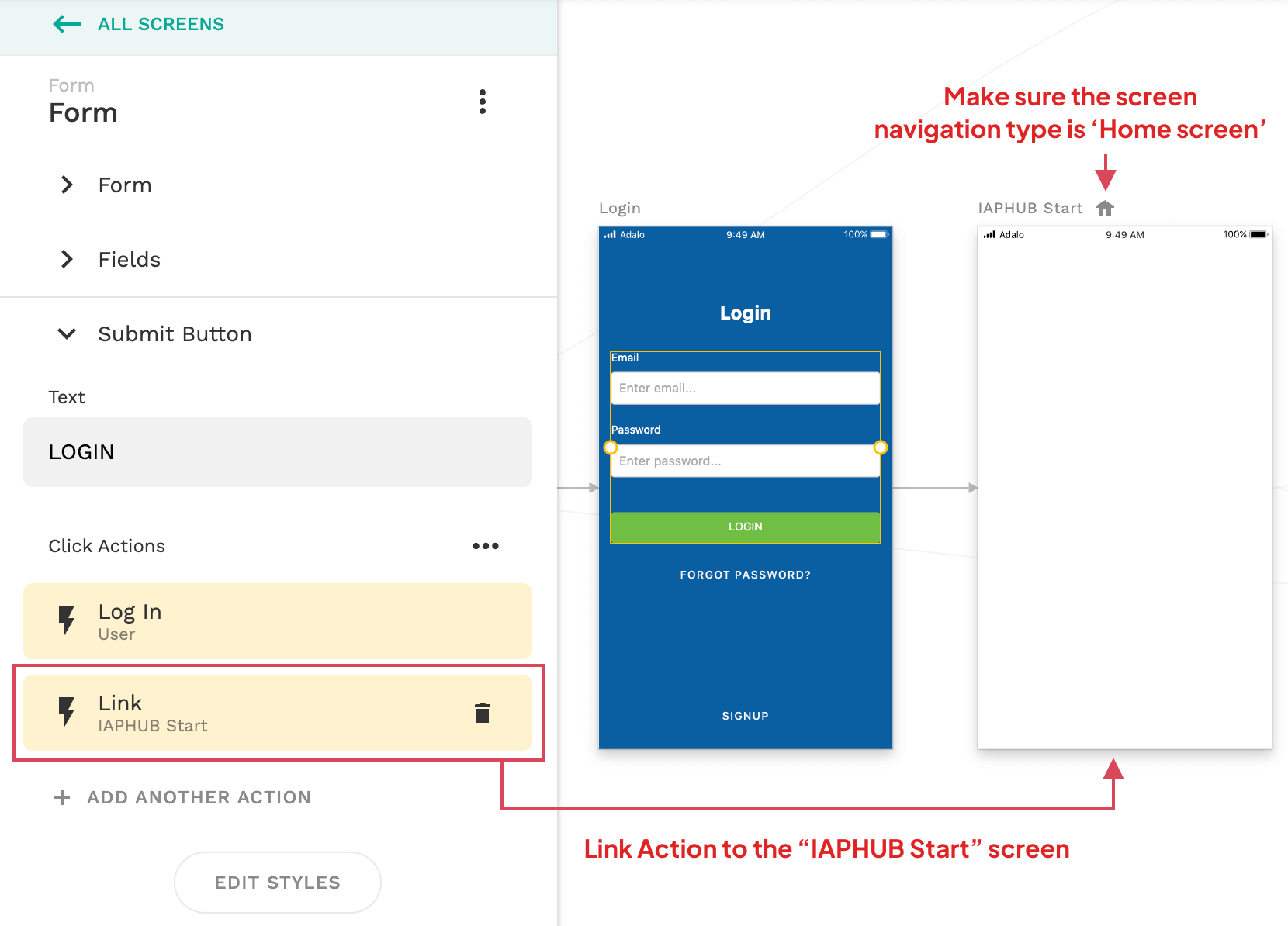This image features a detailed white background with a variety of elements positioned strategically throughout. In the top-left corner, there's a thin rectangular box containing dark green text reading "ALL SCREENS" in all caps, accompanied by a green left-pointing arrow.

Beneath this box is the word "FORM" displayed in black text. Below it, there's a series of tabs labeled respectively: "FORM" at the top, followed by "FIELDS," "SUBMIT BUTTON," and "TEXT" in light gray text. 

Further down, a thin light gray rectangular box with black text inside reads "LOGIN." Under this is more light gray text stating "CLICK ACTIONS." 

Below this section, two pastel yellow rectangular boxes are positioned. The first box features a black lightning bolt symbol with "LOGIN" in black text to the right, followed by the word "USER." The second box, also containing the lightning bolt symbol, displays "LINK," and beneath it, "TAB, HUB, STAR."

Continuing downward, light gray text reads "ADD ANOTHER ACTION" beside a plus sign on the left. Below this is a white oval button outlined in light gray, containing the text "EDIT STYLES" in light gray.

On the right side of the image, several screenshots are aligned. The first screenshot showcases a blue background with a white login screen. The adjacent image on the right is a blank white page.

At the top of the blank white page, red text advises to "make sure the screen navigation type is HOME SCREEN." Additionally, a white arrow from the yellow box labeled "LINK" points towards the blank white page on the right, emphasizing a linkage action. Beneath this, text reads "LINK ACTION to the 'IAP, HUB, STAR, SCREEN.'"